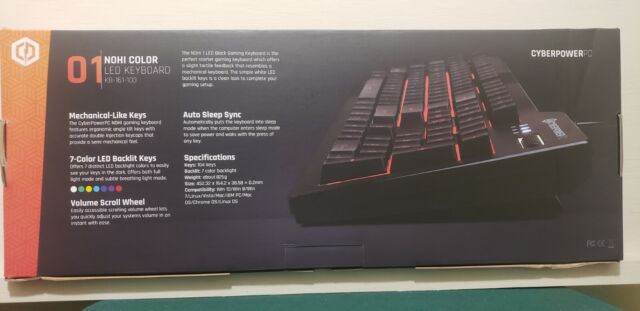This image showcases a NOE Color LED Keyboard. Dominating the left side of the image, there's an orange section featuring a white circular logo followed by the number "01" in orange. Adjacent to this, "NOE Color" is prominently displayed in bold white letters, with "LED Keyboard" written beneath in regular white text. Below these details, the product number is listed. Further descriptions note "mechanical light keys" and "seven-color LED backlight keys," with the colors shown as white, green, yellow, blue, two shades of purple, and red. There are also icons and text indicating features such as volume control, screen scroll wheel, auto sleep sync, and various specifications.

On the right side of the image, a picture of the keyboard is presented. This keyboard is backlit in red, highlighting its black surface and white key labels. The entire background where these details are displayed is black, enhancing the contrast and readability.

In the upper right corner, "CYBERPOWER" is emblazoned in white letters with "PC" in black, suggesting compatibility with Windows PC devices. Lastly, at the bottom, there is a note confirming that the keyboard is FCC regulated.